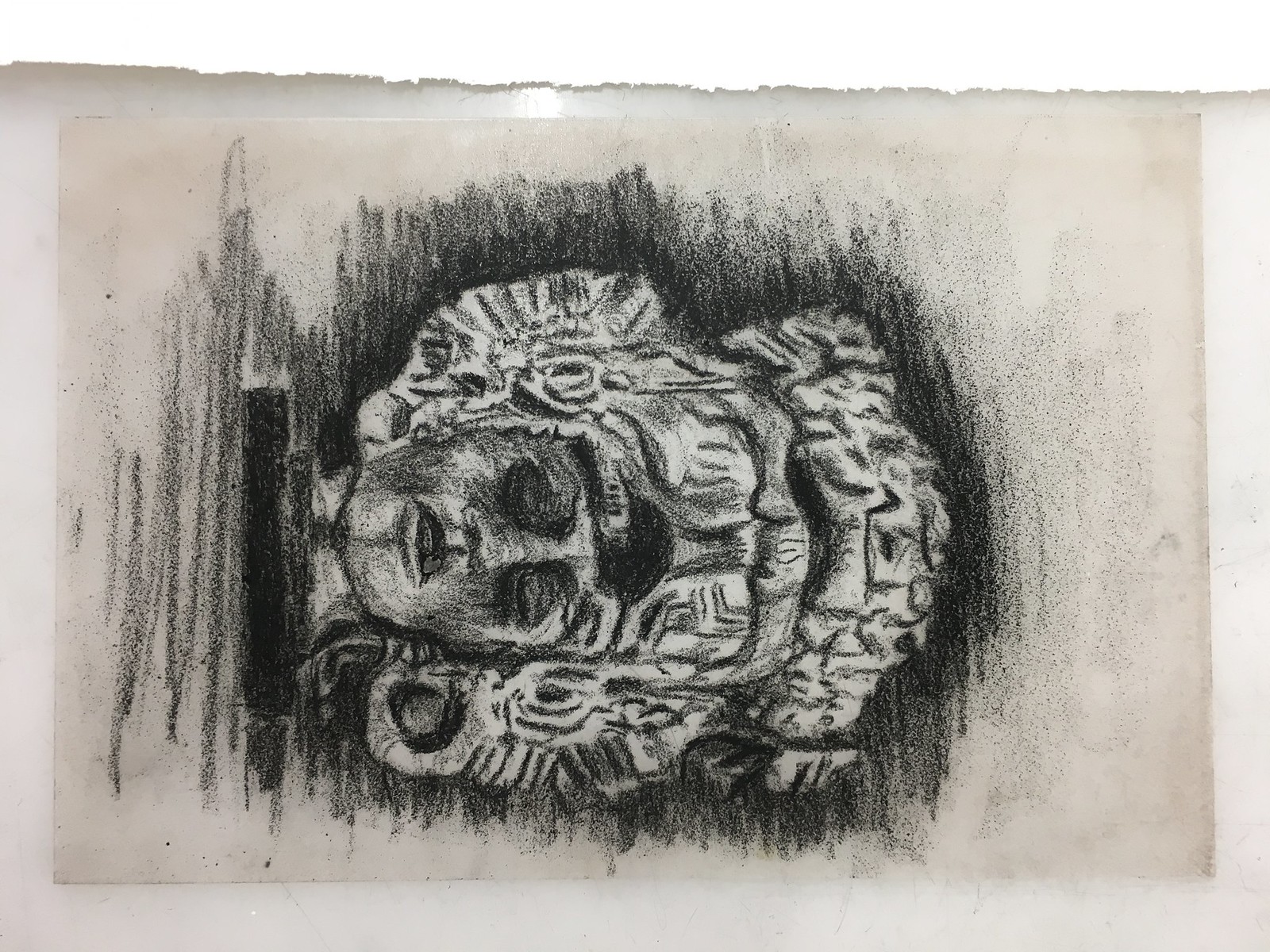The image depicts a horizontally oriented, black and white, charcoal or pencil drawing on a dirt-streaked piece of paper. The artwork shows a side profile of a female face with closed eyes, adorned with eye shadow and slightly parted lips, giving it a haunting, horror-like appearance. The figure wears an ancient-styled headdress, evoking the aura of a Mayan statue carved from stone. The headdress features intricate carvings, possibly depicting animals crawling along the ground. The depiction suggests that the face might be decapitated and is possibly attached to a wooden block for support. The paper on which the image is drawn appears old and dirty, with a torn section at the top, suggesting it has been roughly handled or cropped.